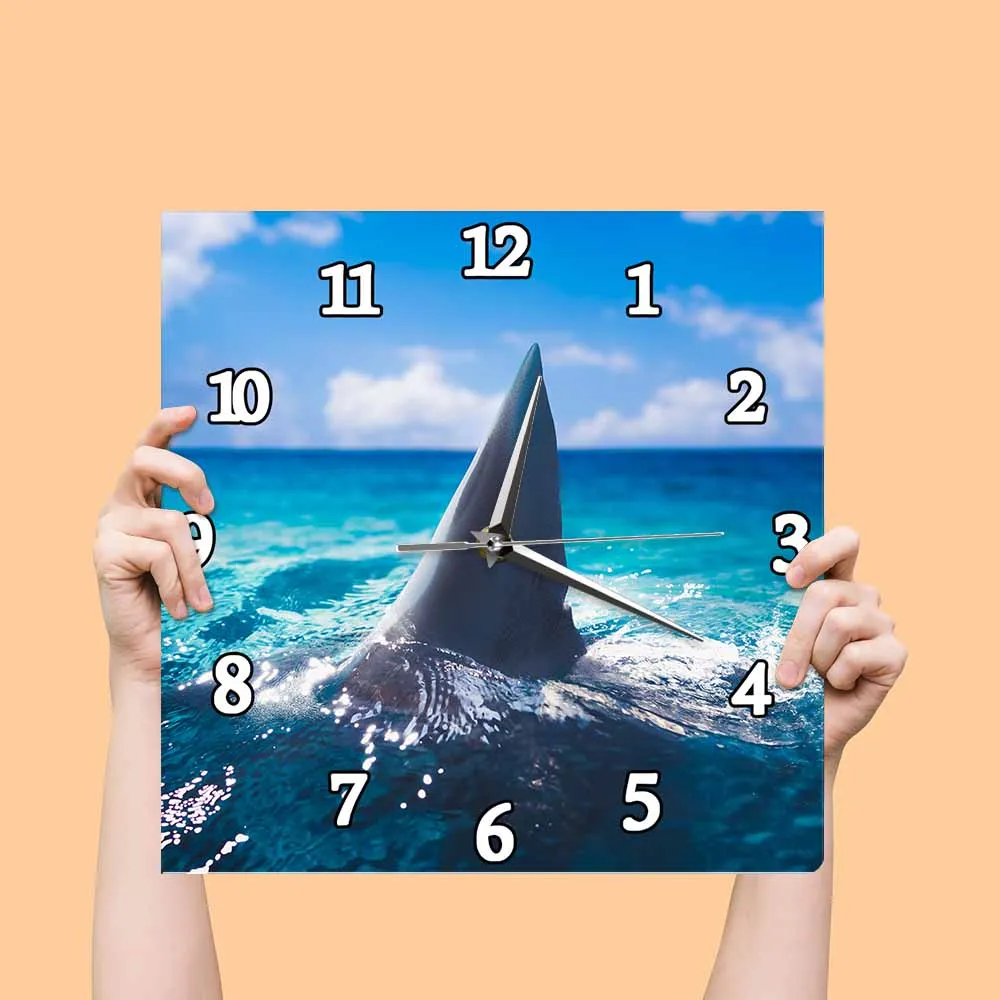In this vibrant image, a pair of hands and arms are prominently featured against a striking pink background. The hands are gently holding a square clock face. The clock face is predominantly blue, vividly depicting the sky and sea, with a whimsical element of a shark's fin emerging from the water, creating ripples and tiny white waves. The clock displays conventional Arabic numerals in white, each outlined in black for clarity, rather than Roman numerals. The clock hands, positioned at 19 minutes past 12, intriguingly extend from the center of the shark’s fin, adding a playful touch to the composition.